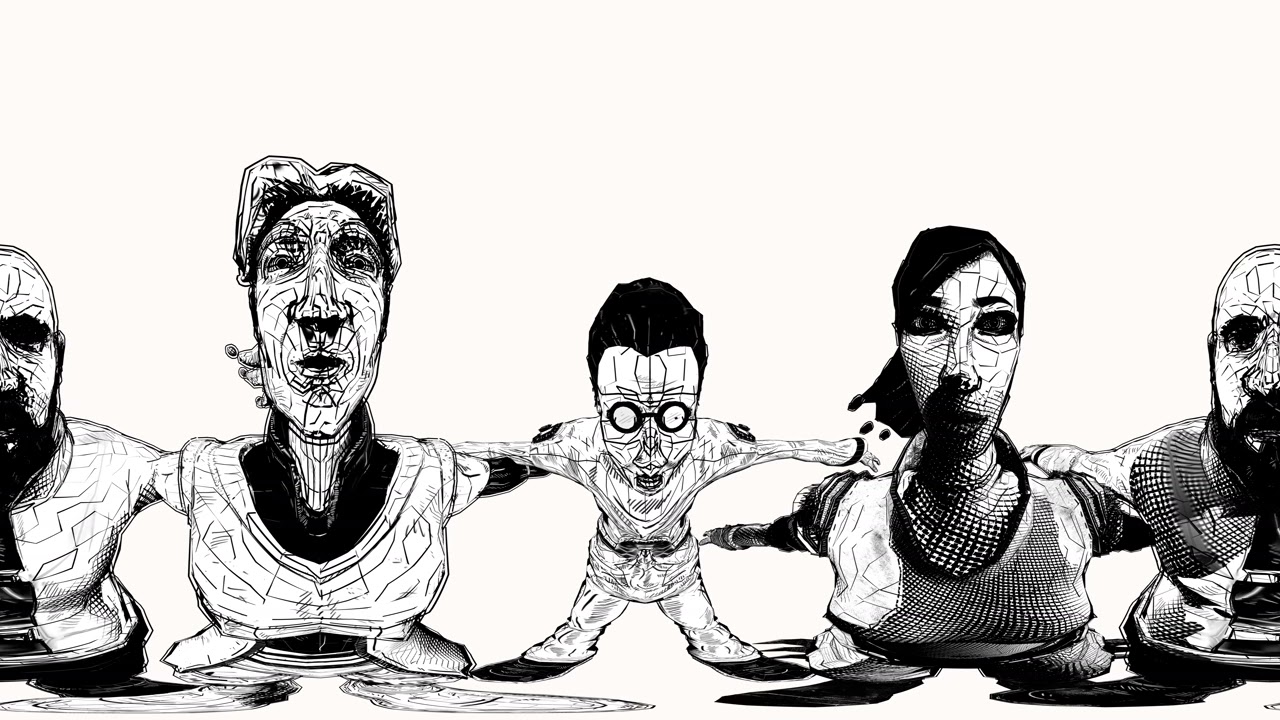In this detailed black-and-white sketch, five distinct characters, rendered with intricate wireframe lines, stand arm in arm in a surreal, almost macabre formation. The central figure appears as a mad scientist with tall black hair and round black goggles, his arms and legs outstretched. To his right, a woman with long black hair and a notably short, stubby torso stands out, her exaggerated features contrasting sharply with the rest. Next to her is a male figure with similar proportions, forming a curious pair. On the far left, two men - one sporting a tie and the other bearing a resemblance to a sinister jester - further emphasize the twisted, caricatured style. Each character's oversized head and distorted body contribute to a dark, edgy aesthetic reminiscent of horror comic art. The meticulous line work and unique, creative design make this drawing an arresting piece of art, blending unsettling elements with a striking visual appeal.